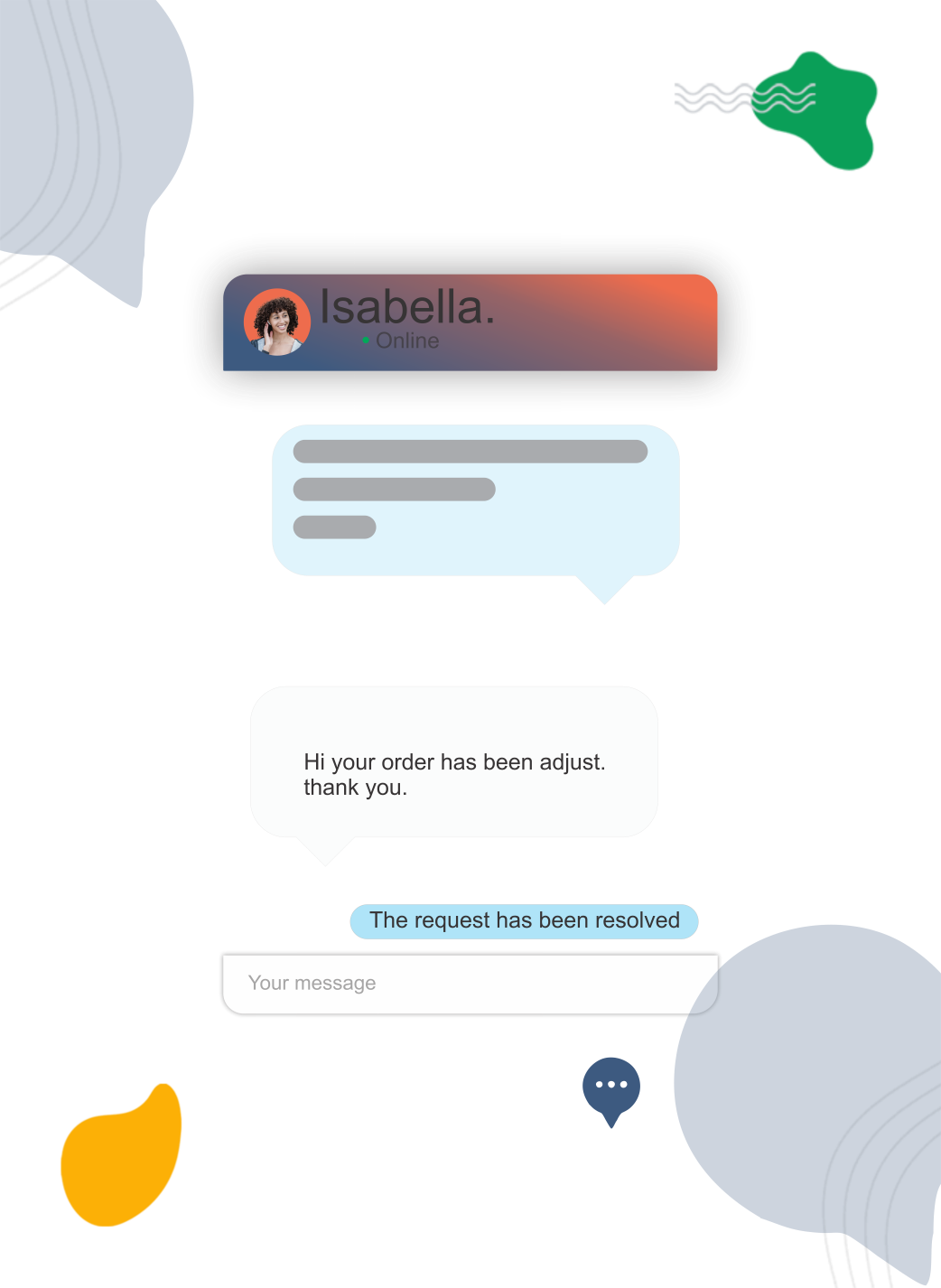In this image, you see a screenshot of a chat page. On the top left, a grey chat design box is visible, while on the top right, there is a green chat design box. At the center, there is a message field displaying a conversation between Isabella and the user. The chat message indicates that Isabella is online and reads, "Hi, your order has been adjusted. Thank you, the request has been resolved." The predominant colors in the image are yellow, grey, orange, green, black, and blue.